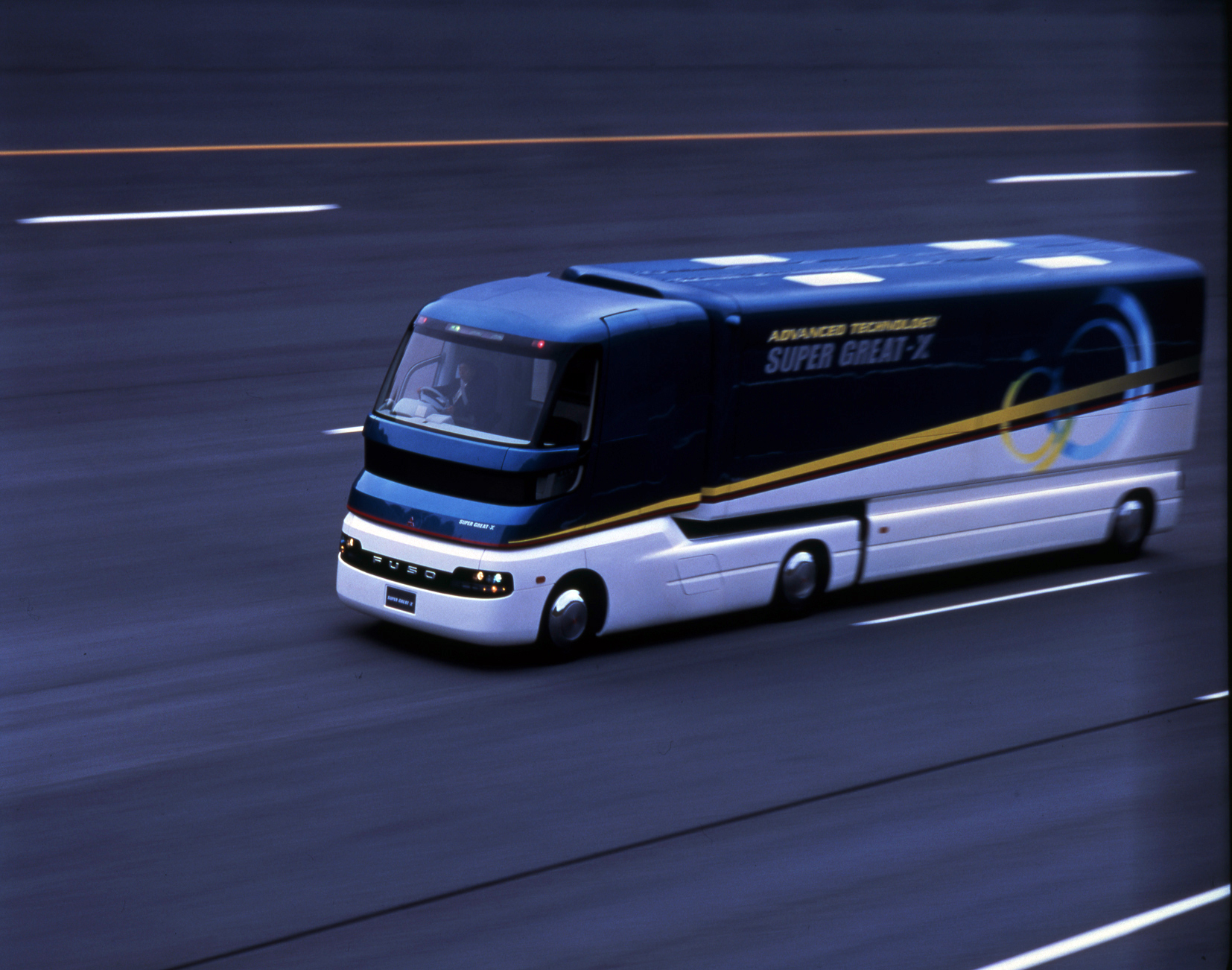The image depicts a vibrant, animated drawing of a bus traveling swiftly along a gray superhighway with at least five lanes of traffic, defined by white and yellow lane markings. The bus appears to be in motion, suggested by the background's intentional blur. Dominating the image, the bus has a striking design with a blue top and cab, black front, and a white lower section. A yellow stripe, reminiscent of a lightning bolt, stretches across the body, complemented by a large blue half-circle arching over the wheels and a white stripe forming a narrow triangle toward the rear. The bus bears the inscription "Advanced Technology Super Great Z" on its side. Chrome-colored wheels add a touch of modernity, and the driver, visible and clad in a blue uniform, is seated at the right-hand side, indicating a European setting. Additional details include four prominent white rectangles on the bus's roof.